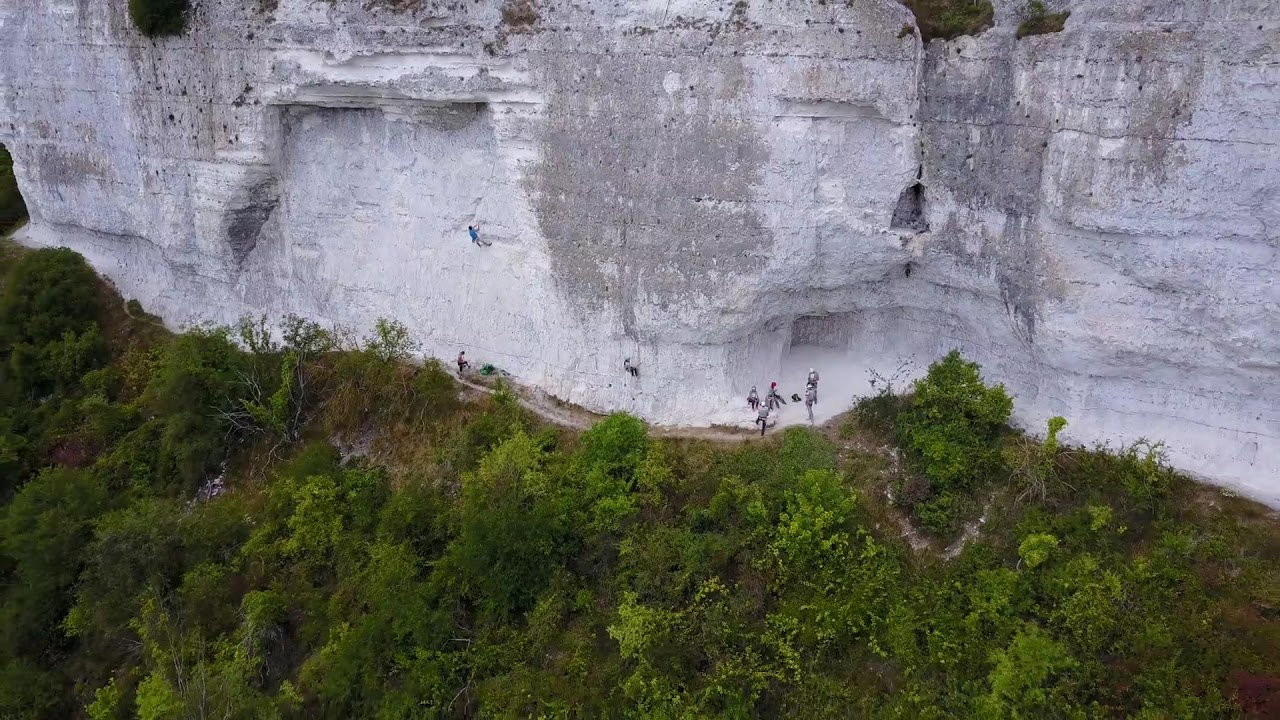This image captures an expansive, rugged landscape featuring a steep white and gray cliff dotted with tinges of greenery at the top. The scene appears to be viewed from either an aerial perspective or from another cliff, providing a sweeping view of the area. At the base of this colossal rock face, dense clusters of trees and bushes abound, alongside a narrow, winding walkway. A few adventurous individuals are visible on the cliff itself; one person is positioned midway up on the left side, while another climber is situated between groups both higher and lower on the face. Additionally, three to four more people are gathered at the middle-right base of the cliff, seemingly preparing for their ascent. The sight of ropes highlights the climbers' activities, underscoring either their upcoming climb or descent. The dynamic composition of greenery and rugged rock set against the backdrop of human determination creates a vivid and detailed depiction of outdoor exploration and adventure.